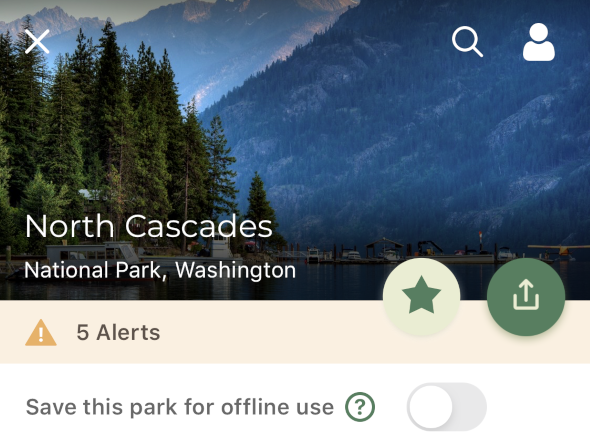Screenshot of a search page for North Cascades National Park, Washington. The background showcases a stunning photo of mountainous hills thick with dense foliage and an expansive forest. Below the hills, a serene lake is visible, bordered by businesses, boats, and tall trees protruding from a land outcropping. Superimposed on this backdrop is the text "North Cascades" with "National Park, Washington" below it. A circular icon containing a star and another adjacent dark green circle with an upward arrow, presumably for uploads, are also displayed. A faint pink banner below indicates "5 alerts" with a triangular caution icon beside it. The white navigation banner underneath reads "Save this park for offline use" accompanied by a question mark icon, and a deactivated slider toggle button for enabling the offline save function.